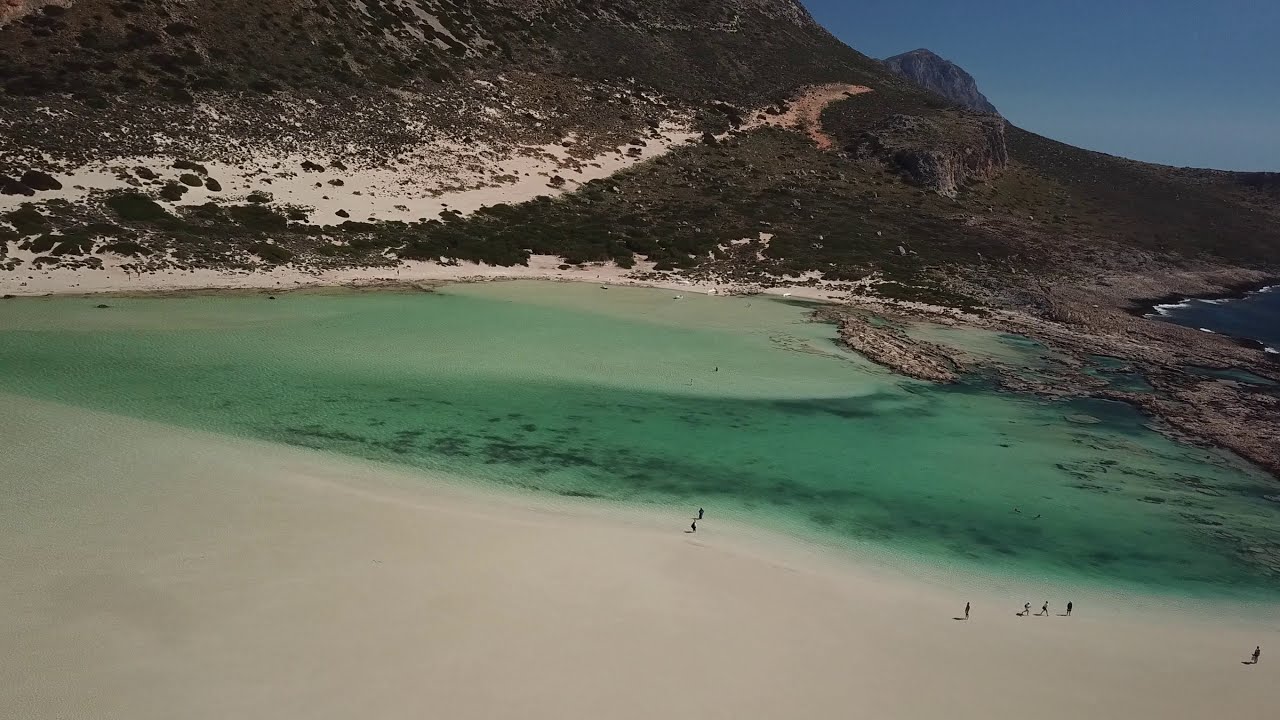The image depicts a remote, secluded beach area characterized by smooth, light brown sand. The horizontal rectangular photograph showcases a striking natural scene featuring brown rocky cliffs with some lighter sandy sections. In the upper left-hand corner, a large cliff slopes downward towards the center-right, where a small, green-hued lagoon-like water body is enclosed between the sand and the cliff. This water varies in color, presenting a bluish-green shade in parts, suggesting shallow depths. The foreground reveals a wide expanse of beach with about eight tiny human figures scattered across, engaging in various activities. The background highlights more sandy dunes and rugged rock formations, while the top right features a distant mountain just touching the horizon under a brilliant blue sky, indicating it is a clear, sunny day.